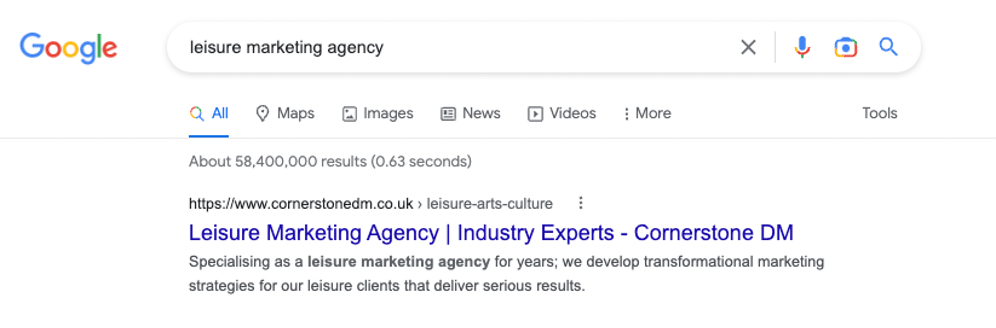A simple screenshot featuring the upper portion of the Google search homepage. The backdrop is predominantly white, with the iconic Google logo positioned in the upper-left corner. Immediately to the right of the logo is the search field, which contains the query "leisure marketing agency." Adjacent to the search field on its right are a series of functional icons: a black 'X' for clearing the query, a blue microphone for voice search, a multicolored camera for visual search, and a blue magnifying glass for initiating the search.

Directly below the search bar is a navigation menu consisting of various search categories. From left to right, these are labeled as All, Maps, Images, News, Videos, More, and Tools, with 'All' selected. Each category is paired with its respective icon: a magnifying glass for All, a location pin for Maps, a photo for Images, a newspaper for News, and a play button within a square for Videos.

Further down, it is noted in gray font that the search yielded approximately 58,400,000 results in just 0.63 seconds. The composition and design elements are minimalistic, emphasizing Google's user-friendly interface.